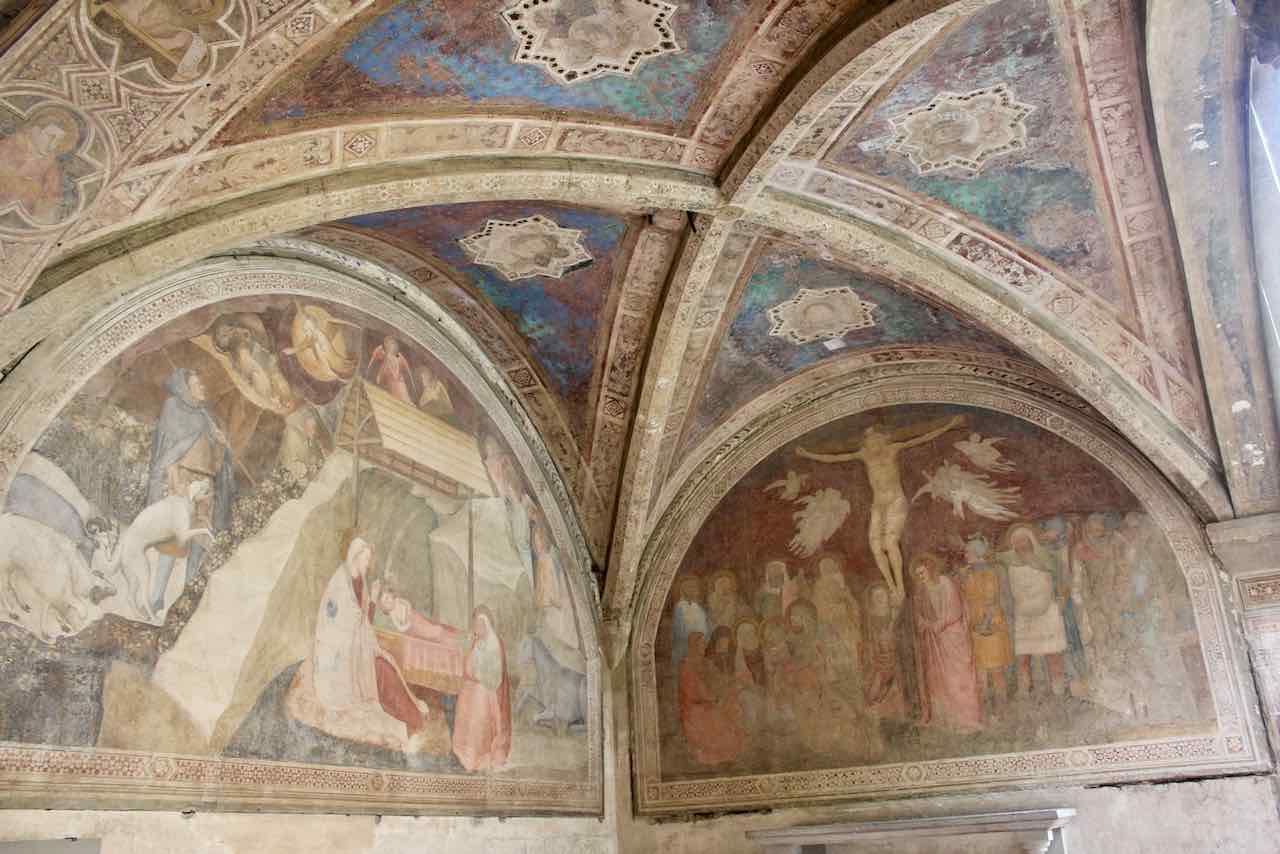The image captures the intricate interior of a cathedral, with an emphasis on the curved, dome-like ceiling and walls adorned with religious artwork. The top of the image reveals beams of light filtering through a window, highlighting the faded yet still vibrant colors of green, purple, and beige that decorate the space. On the right side, there is a striking depiction of Jesus on the cross, with mournful figures beneath him, likely his disciples. The left side features a nativity scene with the Virgin Mary, a child, and surrounding angels. Stars are meticulously drawn on the round ceiling, adding to the celestial and reverent atmosphere. Despite the age and slight fading of the paint, the detailed biblical illustrations maintain their solemn and historical significance, capturing the essence of the sacred space.